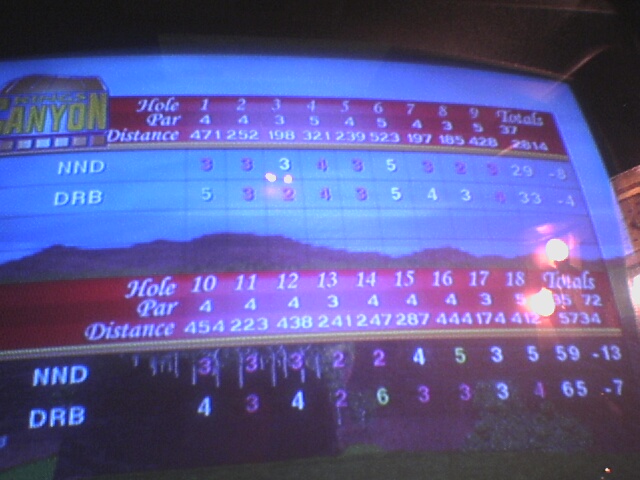The image depicts a low-quality photograph of a screen displaying a golf score menu, with noticeable light glare. The screen shows a digital score sheet set against a backdrop of a golf green, surrounded by trees under a blue sky. Dominating the image are two red horizontal bars. The top red bar features a side menu with headers labeled "Hole," "Par," and "Distance" in white text, accompanied by a series of corresponding numbers, which are tallied up on the right. The bottom red bar mirrors this layout, displaying similar information and totals. On either the top right or left side of the image, the word "Canyon" is visible in yellow block text, likely indicating the name of the golf game or location. The score sheet lists two players, NND and DRB, with their respective scores: NND leads with a score of -13 compared to DRB's -7. Detailed statistics show NND shooting a total of 59 and DRB scoring 65. This organized presentation of data suggests the captured image is likely from an electronic golf game or digital scoreboard.